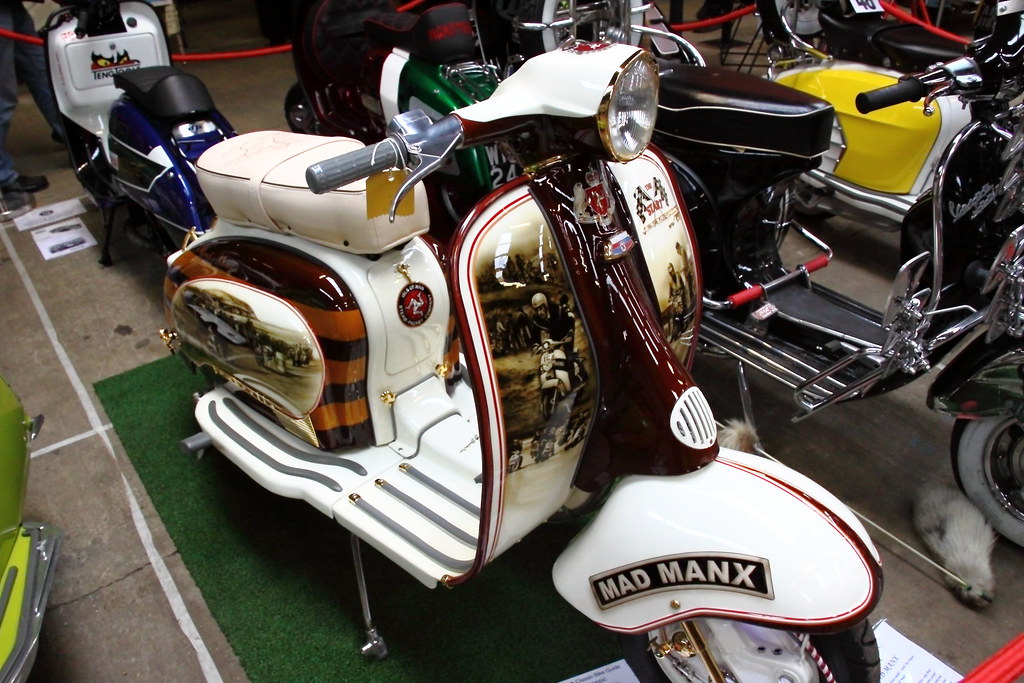The photograph captures a vintage motorcycle exhibition, set in what appears to be a warehouse or garage with a concrete floor and a green faux grass rug underneath the displays. Prominently featured in the foreground is a cream-colored scooter adorned with amber-red and burgundy accents, with the brand name "Mad Manx" clearly visible on the front fender. The scooter is embellished with vintage, shiny printed images and has a white leather seat. Positioned on a green rug, the white footrest adds to its polished, well-maintained look. Surrounding this centerpiece are several other scooters, including a burgundy one and a yellow and white model visible in the upper left corner, along with blue and green-colored scooters in a row behind. Tape on the concrete floor delineates the parking spaces, contributing to the showroom-like atmosphere. People stand behind a red line in the background, suggesting these meticulously displayed scooters, complete with informational paper sheets underneath, are part of a well-organized motorbike showcase.